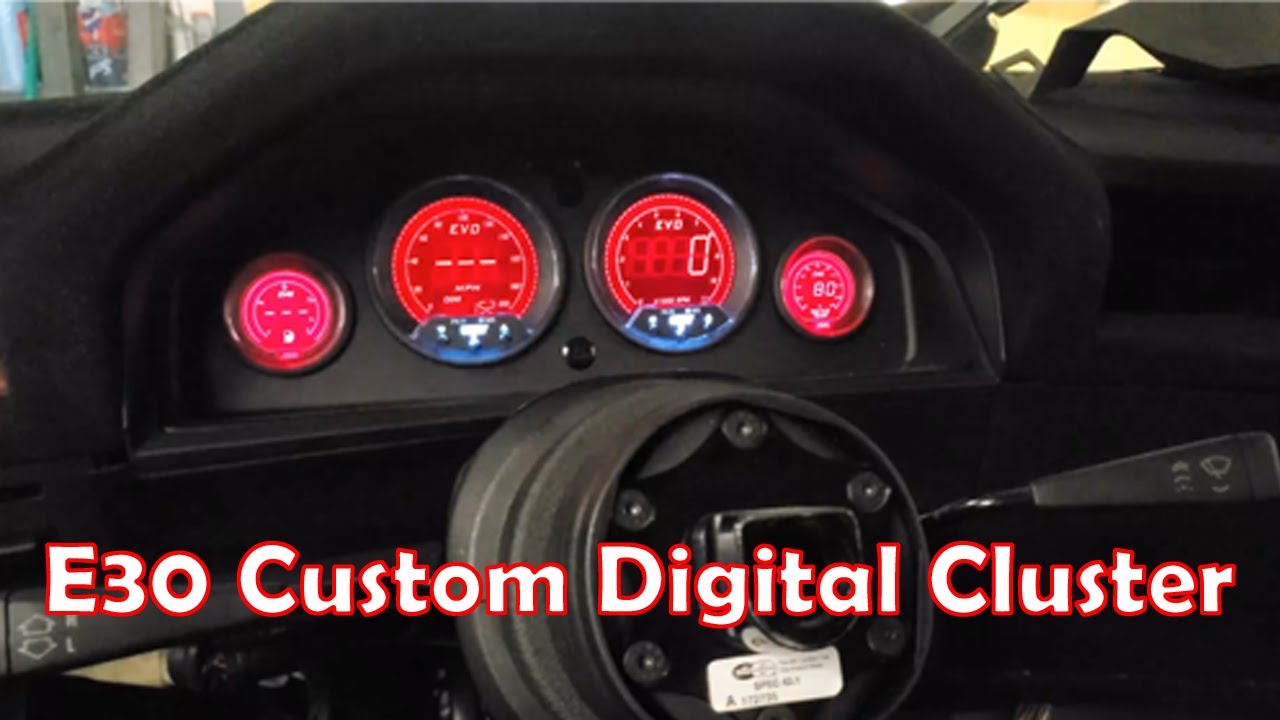This image is a close-up of a car's digital dashboard, specifically labeled "E30 Custom Digital Cluster" in white text outlined in red. The dashboard is predominantly black with four brightly lit gauges. The two larger gauges in the center and the smaller ones on the outer edges are primarily red with white numbers, featuring a mixture of fuchsia and pink tones. These gauges include readings for fuel, speed, and oil. Below the gauges, there's a modern, round metallic black wheel, which is not a steering wheel, hinting at a specialized machine or an older type of car. The background and surroundings of the dashboard are matte black, lending a sleek, high-quality appearance. Notably, there is a small blue area beneath the two central gauges. The absence of a steering wheel and the detailed setup suggest this image might be part of an advertisement or promotional material for custom car modifications.